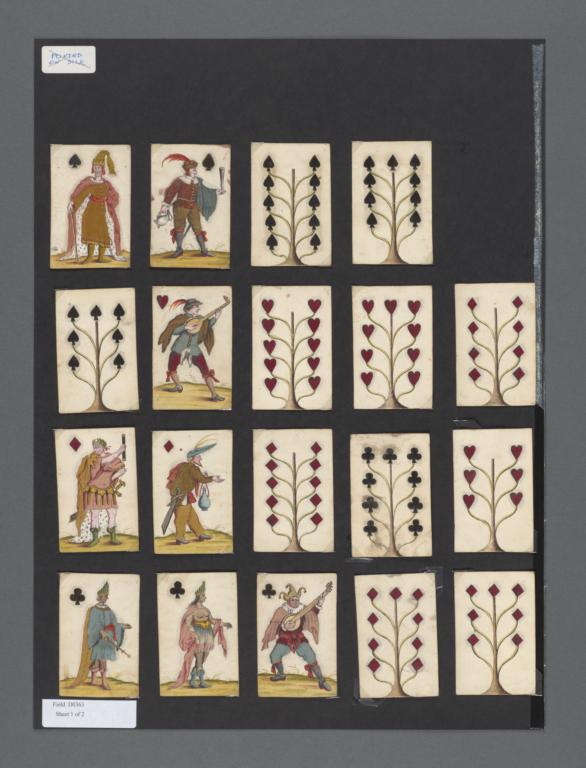This image depicts an antique, possibly hand-painted collection of playing cards displayed in a rectangular, portrait-oriented frame with a dark gray border and a black background. The cards are meticulously arranged in a grid format: four columns and four rows, except the top row, which has only three cards. 

The cards feature elaborate illustrations of medieval figures and suits. The top row showcases spades, with the first card depicting a person dressed in an ochre-colored robe. The second card in the row shows a figure wearing brown pants, a collared shirt, and a feathered hat. The third card in this row displays a tree where the branches end in spades, indicating various quantities. 

The subsequent rows follow a similar pattern but with different suits: hearts, diamonds, and clubs. Each of these rows includes cards with characters dressed in medieval attire and intricate designs. Notable among the illustrations are character cards such as the King, Joker, and Jack, each prominently featuring their designated suit symbols. The cards are distinctly old, suggesting that this is a historical or antique collection. The bottom of the frame includes a label, though it is not legible in the image.